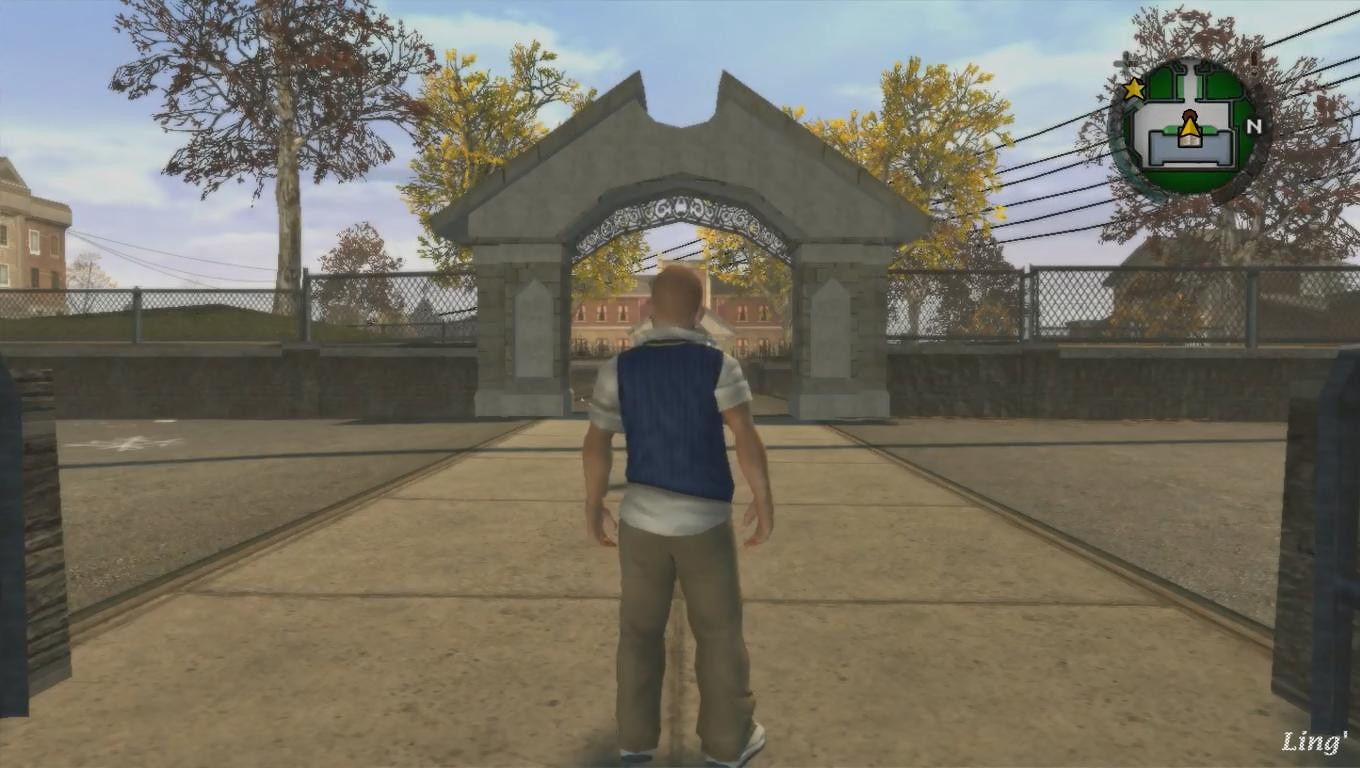The image is a scene from a computer game featuring high-quality graphics. It depicts an outdoor setting where a man with a crew cut, who appears to be white, stands on a sidewalk facing a grand entranceway. He is dressed in khaki pants, a white shirt with the sleeves rolled up past his elbows, and a blue light vest. The entranceway, which has a large arch, could potentially lead to a boarding school, an old-fashioned insane asylum from the 1930s, or a wealthy estate. On either side of the arch, there is a low stone wall topped with a fence, behind which large trees and green grass are visible. Directly ahead beyond the arch, there is a brick building. In the right-hand corner of the image, there is a symbol featuring a green center, white surrounding it, and accents of yellow, with an "N" on the right side. The sky above the scene is blue, adding to the serene yet mysterious atmosphere of the setting.